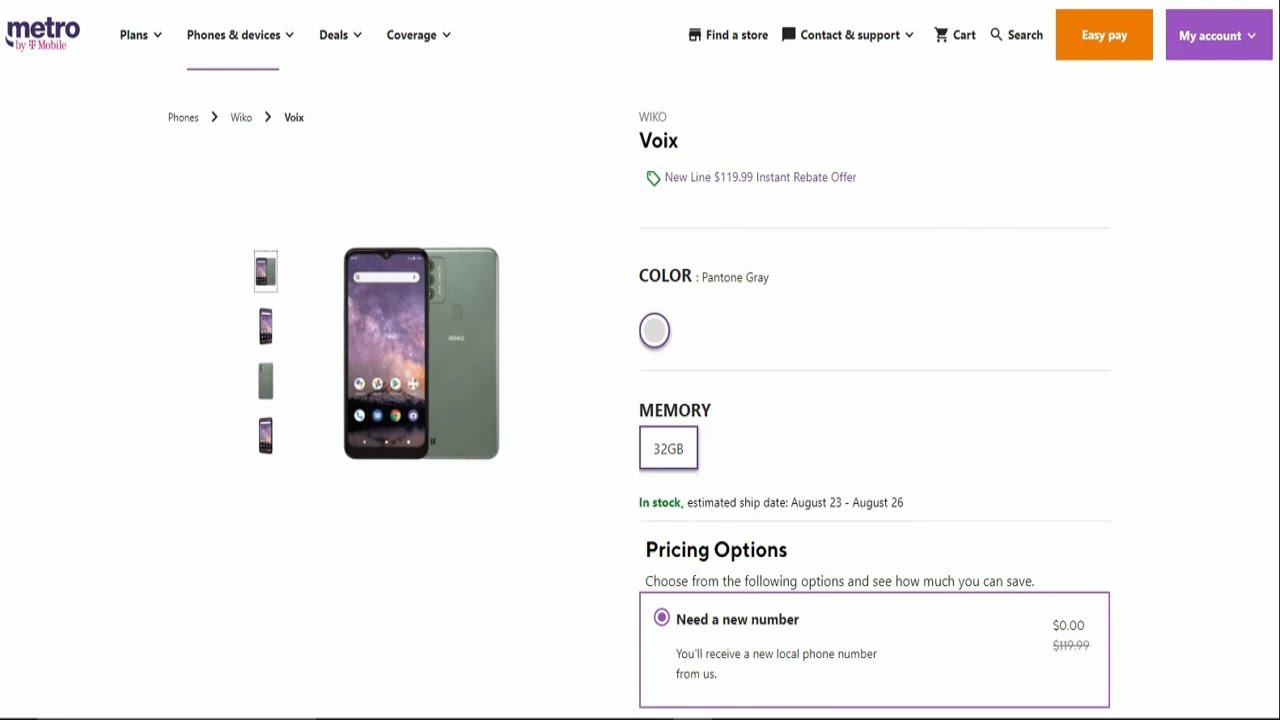In this image, the top left corner features the "Metro by T-Mobile" logo. To the right of the logo, there are four navigation categories: "Plans," "Phones & Services" (underlined), "Deals," and "Coverage." On the far right side, there are additional categories: "Find a Store," "Contact & Support," "Cart," and "Search." 

Next to these, there are two squares: an orange square labeled "EasyPay" and a light purple square labeled "My Account." Beneath these elements, the text "VOIX" is prominently displayed.

The lower part of the image showcases a cell phone. The phone screen is purple, while the back side is gray. To the right of the phone, there's a representation of the available color, depicted as a purple circle shaded with gray. Below this, "32 GB" is displayed within a square, indicating the phone's memory capacity. Further down, the status "In Stock" and the ship date are mentioned. 

Below this section, there are pricing options in bold black text accompanied by a suggestion in gray text to "choose from the following options and see how much you can save." The option "Need a new number" is highlighted with a light purple rectangular outline, showing a total cost of "$0.00."

A thin black line marks the bottom and right side of the image, serving as an outside barrier. The entire background of this image is consistently white.